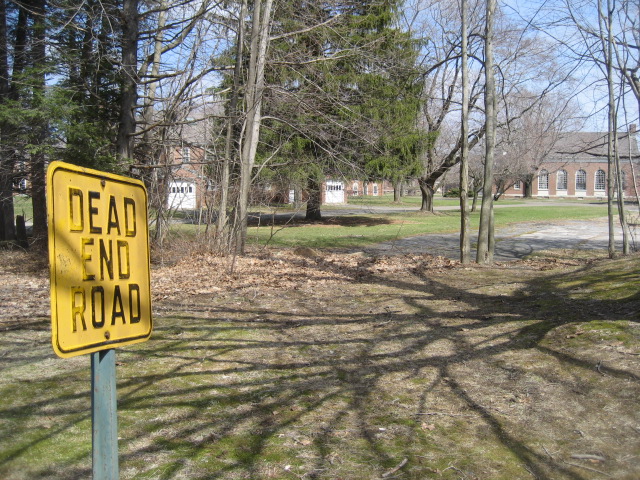This outdoor photograph captures a rustic scene featuring a mix of natural and man-made elements. Dominating the center foreground is a gravel pavement with patches of green grass poking through, leading the eye towards two primary buildings in the background. One building, likely a brown brick church given its characteristic windows with square panels but no stained glass, stands prominently alongside another structure, probably two houses identified by their two-car garages and grey roofs. Interspersed among these buildings are numerous trees, some lush with green leaves while others are starkly bare, adding a contrast of life and dormancy. On the left side of the image, a silver pole displays a weathered yellow "Dead End Road" sign with faded black text, rooting the scene in a subtle sense of closure and tranquility. Above, the sky peeks through, a light blue expanse that complements the earthy tones below.